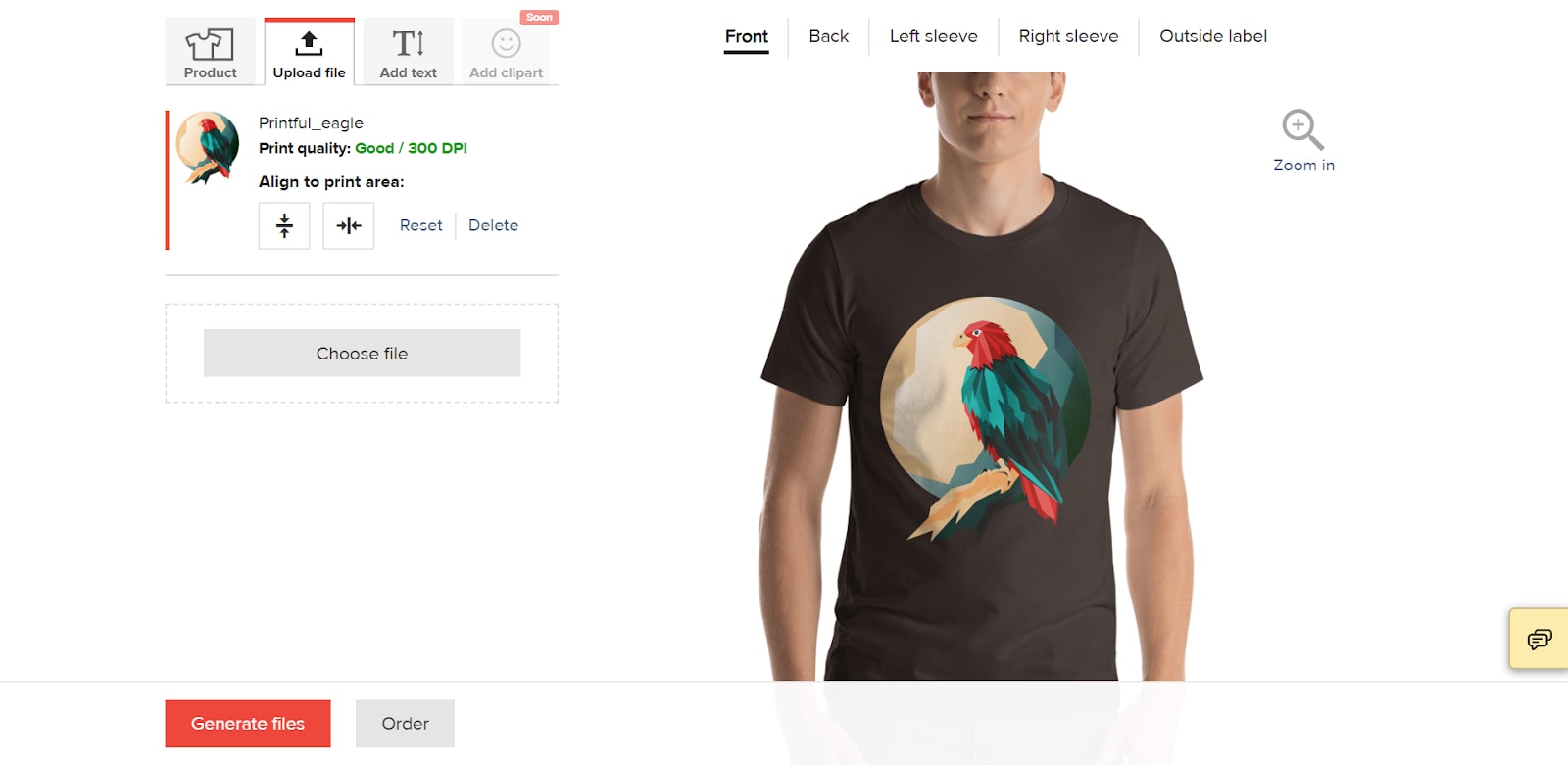The image is a screenshot from a website, specifically showing a product customization interface. The interface appears to belong to Printful, as indicated by the label "Printful_eagle." Notably, the print quality is marked as good, and it aligns well with the designated print area.

Prominently, the screen displays a front view of a male model, identified as Caucasian, wearing a brown t-shirt. The t-shirt's front features a sizable circular graphic. Within this circle, a vibrant bird illustration is presented, showcasing a bird with green and red plumage perched on a brown branch. The circle encompassing the bird is adorned with tan, brown, and green hues.

At the top of the interface, there are options to upload a file or add text to the design. Additional views of the t-shirt are accessible, permitting users to inspect the back, left sleeve, right sleeve, and outside label. These options help ensure a comprehensive view of the custom design.

Near the bottom of the screen, there are functional buttons to generate files, highlighted in orange, and place an order, presented in light gray. On the lower right, an image with a tan background features two overlapping message bubble icons, though their exact purpose remains unclear. The entire interface is set against a clean, white backdrop, designed to enhance user focus on the customization process.